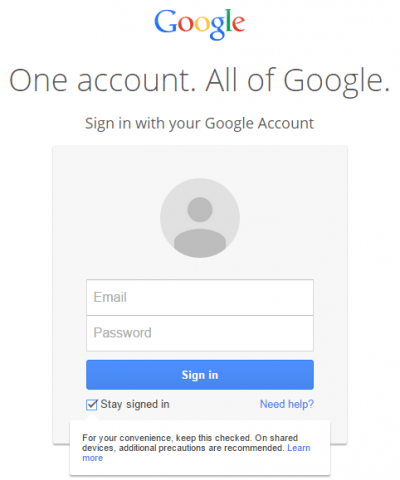This screenshot captures the Google sign-in page, prominently featuring a clean and minimalist design with a white background at the top. Centered at the top is the unmistakable Google logo, showcasing both G's in blue text, the first O and the E in red text, the second O in yellow text, and the L in green text.

Directly beneath the logo, in the largest font on the page, is the tagline: "One account. All of Google." Below this, in slightly smaller text, the instruction "Sign in with your Google Account" is displayed, guiding users toward the sign-in process.

A light gray rectangle dominates the center of the page. At the top of this rectangle is a large circle with a slightly darker gray background, within which resides a generic image of a person rendered in gray.

Two input fields are positioned beneath this circle: the first is labeled "Email" and the second "Password." Below these fields is a blue rectangular button, centrally aligned and bearing the white text "Sign In."

In the lower left corner, a small checkbox with a checkmark beside the text "Stay signed in" offers users the option to remain logged in. Opposite this, in the lower right corner, the blue text "Need help?" provides a link for additional assistance.

Further enhancing user convenience, a white box adjacent to the "Stay signed in" checkbox includes the advisory: "For your convenience, keep this checked. On shared devices, additional precautions are recommended." This is followed by a "Learn more" link in blue text, inviting users to find out more information.